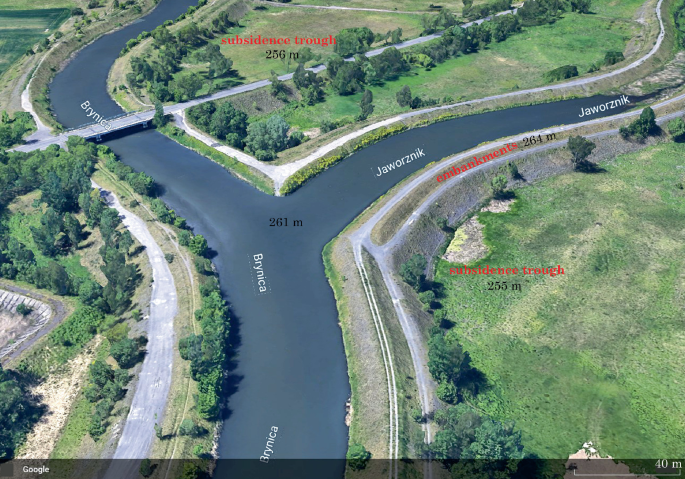The detailed image is an overhead, landscape-oriented map showcasing a bifurcating roadway or river, possibly viewed from a high altitude or generated by AI. The main roadway, labeled Bryneika, originates at the bottom center and splits into a Y-shape, continuing as Bryneika to the left and morphing into Jaworsnik to the right. The image, potentially a Google Maps capture, features lush greenery with trees and grassy areas on both sides of the split. Notable landmarks include roads, bridges crossing the left split of the river, and several instances of labeled subsidence troughs and embankments, indicating detailed land measurements such as "subsidence trough 256 meters" and "embankments 264 meters." Additionally, the image provides a key scale of 40 meters for distance reference, enhancing its practical utility.